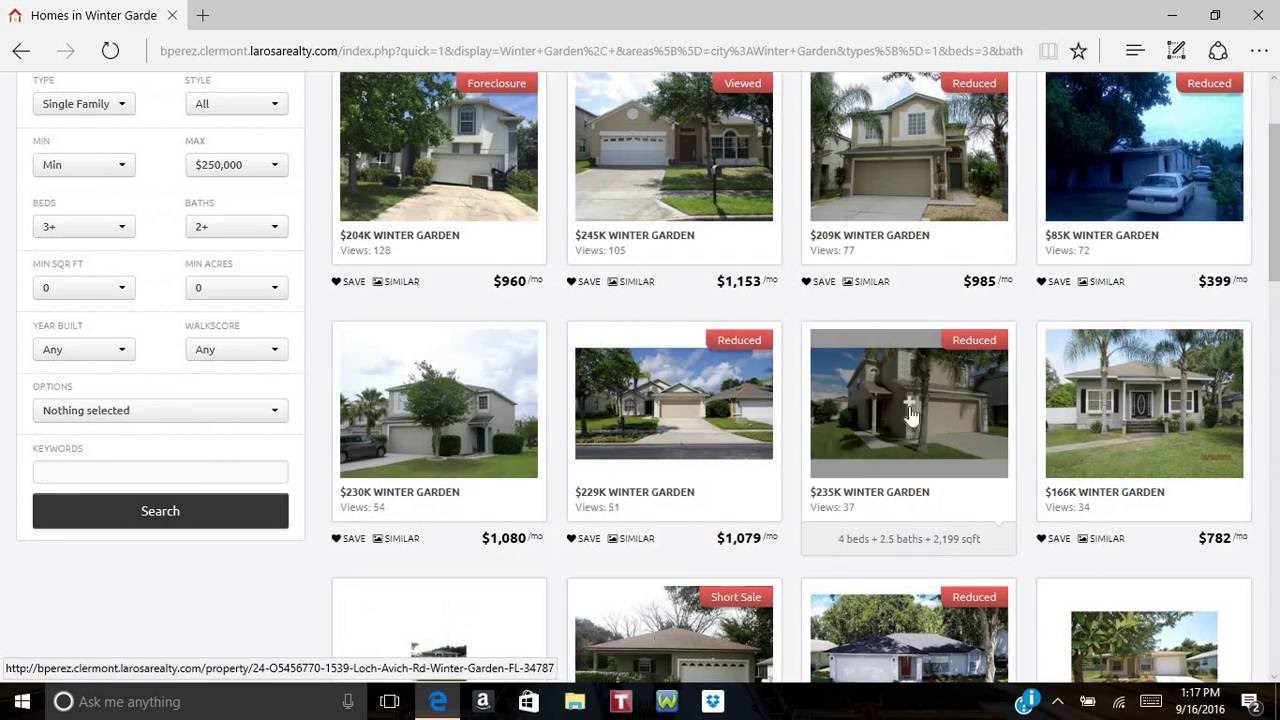This screenshot showcases the search page of the Laros Realty website. The left quarter of the page features a grid of search options arranged in a two-column, five-row format. Each of the drop-down boxes is a light shade of gray, providing various filtering criteria. The rows offer the following selections:

1. **Type and Style:** General categories for the property.
2. **Minimum and Maximum Price:** With the minimum price currently set to 'Min' and the maximum price set to $250,000.
3. **Beds and Baths:** Set to '3+ beds' and '2+ baths', respectively.
4. **Minimum Square Feet and Minimum Acres:** Both set to zero.
5. **Year Built and Walk Score:** Both set to 'Any'.

Below these are rows for additional options and a keyword search bar, alongside a prominent black "Search" button with white text.

The remaining three-quarters of the page display a 3x4 grid of property listings. Each listing predominantly shows the front view of a single-family home, set in what looks like a tropical environment, possibly Florida. Homes vary between single and double-story structures, featuring garages, driveways, and assorted landscaping.

Each property in the top row has a red box in the upper right corner indicating special statuses: "Foreclosed," "Viewed," "Reduced," and "Reduced." The other rows have labels such as "Reduced" and "Short Sale" for certain properties, while some lack special indications.

At the bottom of the screenshot, the typical Windows interface is visible with a black taskbar including a visible time of 1:17 p.m. and date of 9-16-2016. The Microsoft logo and Cortana search bar with a voice icon are present on the left. The browser in use is Microsoft Edge, with the tab title reading "Homes in Wintergard."